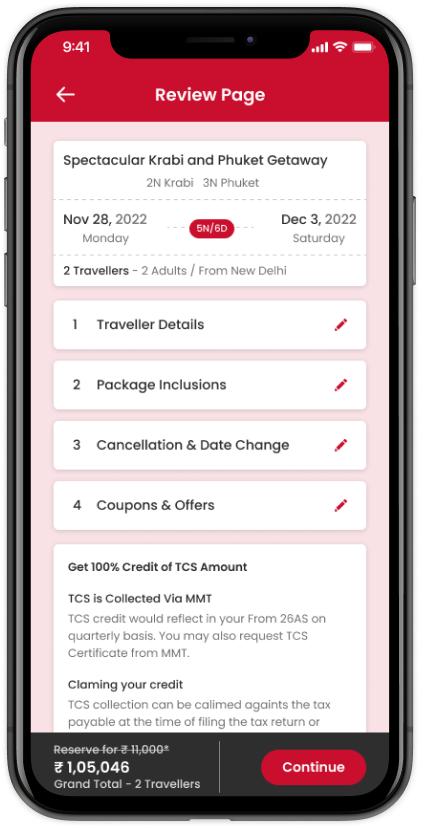This image is a screenshot of a mobile phone displaying a travel booking application interface. The phone's frame is visible around the edges of the screenshot. At the top, there is a red rectangle with a cut-out for the front camera, housing the time displayed in white in the upper left corner, and the reception, Wi-Fi, and battery symbols in white on the right.

Below the top bar, a white left-pointing arrow is centered on the screen, accompanied by the text "Review Page." The background transitions to light pink, featuring six white rectangles with various texts. 

The top rectangle displays text in black, reading "Spectacular, Crabby, and Funk It Getaway," with some smaller gray text below. Further down, centered on the screen, is a red button. To the left of this button, it says "NOV 28, 2022" and to the right "DEC 3, 2022," with "Monday" beneath November 28 and "Saturday" beneath December 3.

Below these dates, on the left-hand side, black text reads "2 travelers - 2 adults / from New Delhi." This is followed by four consecutive white rectangles with headings and red pen icons on the right:
1. "Traveler Details" with a number "1" and a red pen icon.
2. "Package Inclusions" marked as number "2" with a red pen icon.
3. "Cancellation and Date Change" under number "3" with a red pen icon.
4. "Coupons & Offers" labeled as number "4" with a red pen icon.

The subsequent section has a prominent statement in black, "Get 100% Signed Credit of TCS Amount," with the note "TCS is collected via MMT" beneath it. Below, there are three lines of light gray text detailing the process of claiming your credit, though only the first two lines are fully visible, the rest slightly cut off.

Finally, in the bottom right-hand corner, a red "Continue" button is prominently displayed.